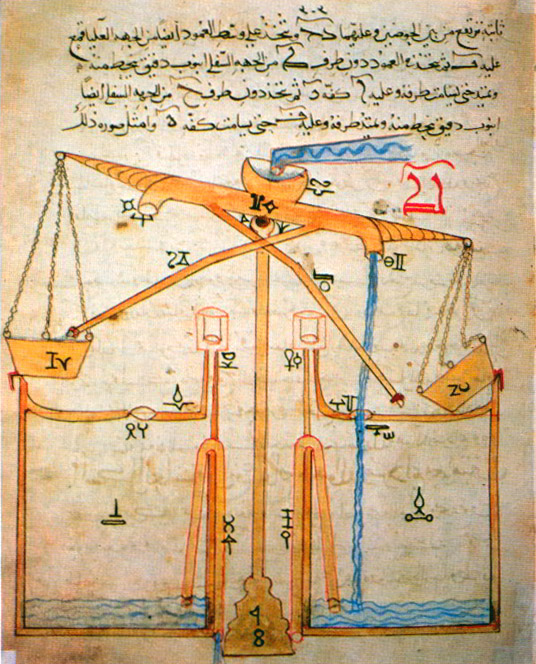This detailed, hand-drawn image depicts an intricate, ancient machine, possibly from an older era, designed to distribute water. The drawing resembles a blueprint or schematic diagram, showcasing how water is poured into a bowl-like top, then flows through a network of orange pipes and spouts to various locations, eventually filling reservoirs at the bottom. The water is illustratively colored red. The machine, evocative of old-time inventions, appears intended to showcase the mechanics of water distribution or a fluid pumping system, akin to the scales of justice with baskets. The scale has one basket marked with "IV" and another with "ZU," both tilted, and connected by three chains to the top of the apparatus. All around the machine, there are handwritten labels in black ink, resembling hieroglyphics, which, along with the four lines of Arabic text at the top, add to the drawing's archaic feel. The entire image rests on a background that mimics aged paper or papyrus.